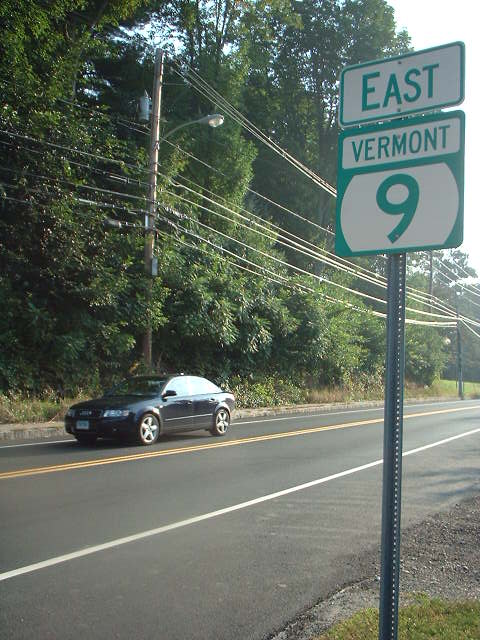A daytime photograph captures a quiet stretch of road marked by yellow center lines and white outer edge lines. Prominently positioned on the right side of the image is a road sign that reads "East Vermont 9." On the left side, opposite the sign, utility poles stretch along the roadside, adorned with power lines. One of the poles features a single, unlit street light. The background showcases dense trees and overgrown brush, adding a touch of wilderness to the scene. In the foreground, a dark blue or dark green sedan, likely an Audi, approaches the camera, adding a dynamic element to the otherwise static landscape.